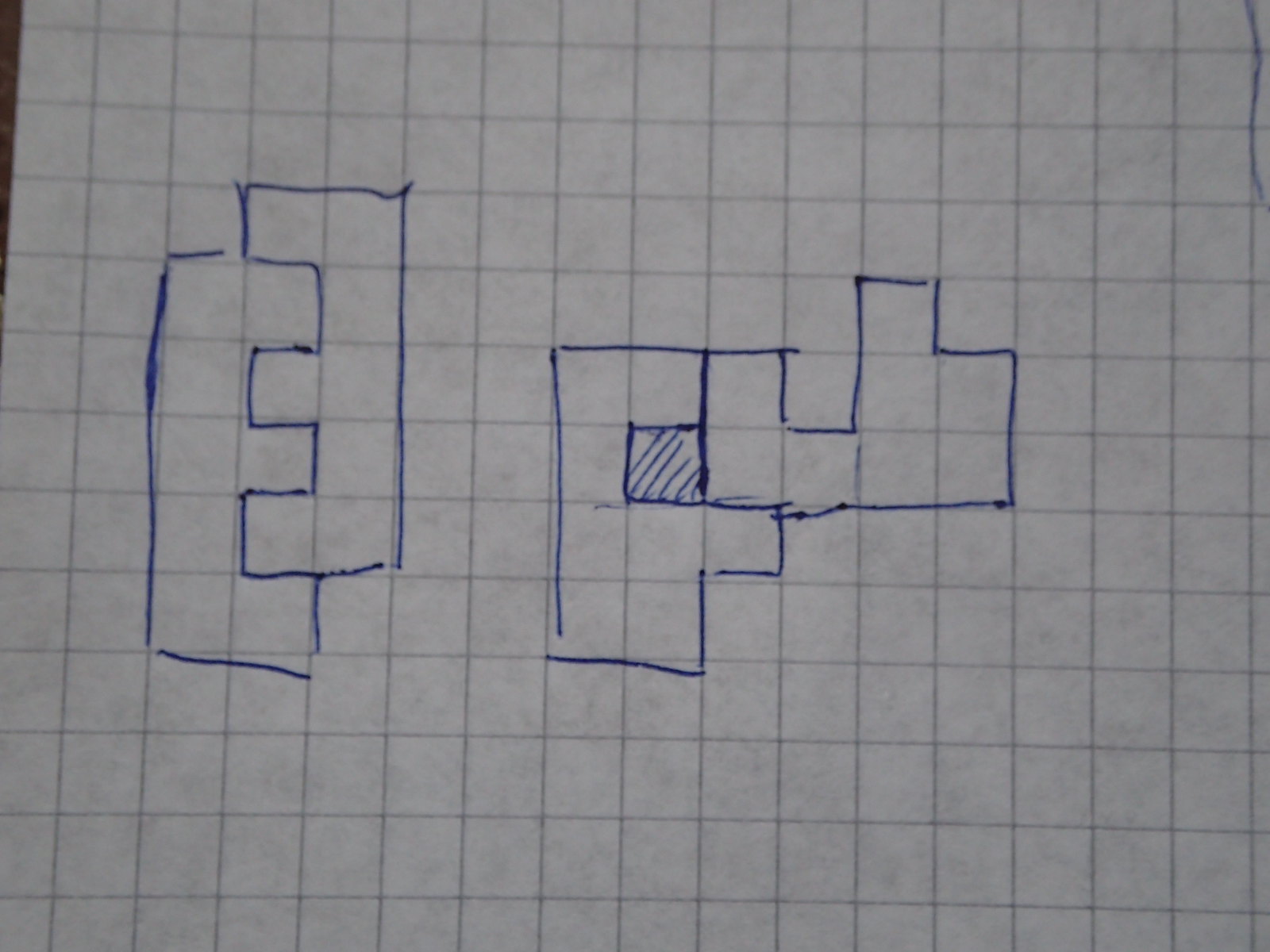This photograph captures a piece of graph paper with various blue pen markings, taken indoors under suboptimal lighting conditions, likely from an overhead light. The graph paper, while originally white, appears greyish due to the poor lighting, with its grid lines rendered in light grey.

On the left side of the image, a capital 'E' has been meticulously drawn in bubble writing. This 'E' is outlined to be two blocks wide and five blocks high, with an inventive overlay of an inverted 'E' resembling a backward number three, seamlessly fitted inside the original 'E' like interlocking teeth.

At the center of the image, one square of the graph paper has been specifically outlined and shaded using diagonal lines. Surrounding this shaded square is an abstract shape, drawn with the same blue pen, adding an element of intrigue to the overall composition.

Towards the top of the image, another enigmatic shape lies on its side, resembling unconventional Tetris pieces randomly placed on the paper. These additional shapes lack a clear form or purpose, contributing to the irregular and experimental aesthetic of the drawing.